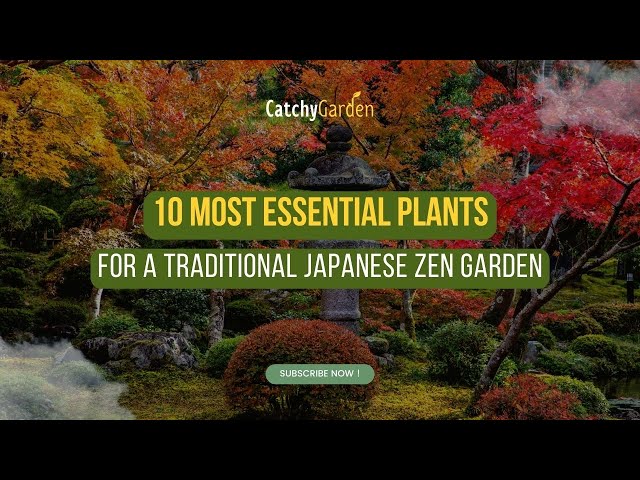The vibrant advertisement for a gardening or horticulture magazine displays the title "Catchy Garden" prominently across the top center in white lettering, with the words "10 Most Essential Plants for a Traditional Japanese Zen Garden" just below it in capitalized golden yellow and white letters, contrasting against a solid green background. The vivid background image features a serene Japanese garden, filled with a diverse array of Japanese maples and shrubs that transition in color from yellow to orange, green, and a particularly striking red. Central to this tranquil scenery is a stone statue with a grayish, misty appearance, reminiscent of traditional Zen garden ornaments. The ground is covered in lush green moss and flanked by rounded shrubs, with a notable dark red shrub positioned beneath a prominent "Subscribe Now" button at the bottom, suggesting an interactive feature, possibly for a digital magazine or online content subscription. The scene is highlighted by scattered rocks adorned with green moss, and a touch of atmospheric fog adds to the peaceful ambiance.